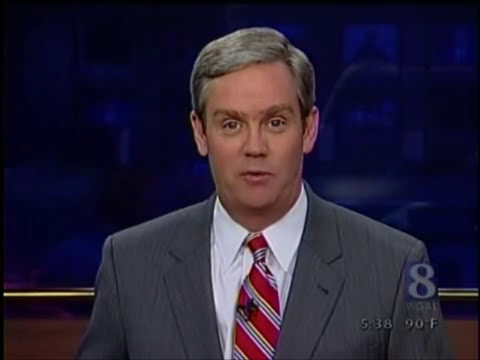This detailed image capture is a still shot of a news broadcast showing a middle-aged, clean-shaven Caucasian male news anchor, roughly 45 years old, wearing a gray suit jacket, a white collared shirt, and a distinctive red tie with diagonal stripes of purple and yellow adorned with symbols. His gray hair is neatly parted on the right side, and he has raised brown eyebrows. Both of his ears are visible. The anchor is looking directly into the camera, with a microphone clipped to his tie, indicating he is speaking to the viewers. 

The background of the image consists of a dark blue, mottled screen with various light spots, creating an out-of-focus effect in the top two-thirds of the frame. Below this is a horizontal strip comprising two wood-tone bands, the top one lighter brown and the lower one darker brown with a gold line running through it. 

On the bottom right corner of the image, the logo for Channel 8, possibly WGAL, is prominently displayed. Next to the logo, the time reads either 5:18 AM/PM or 5:38 AM/PM, and the temperature is shown as 90 degrees Fahrenheit. The image captures the essence of a standard local news broadcast, framed tightly to focus on the anchor delivering the news.